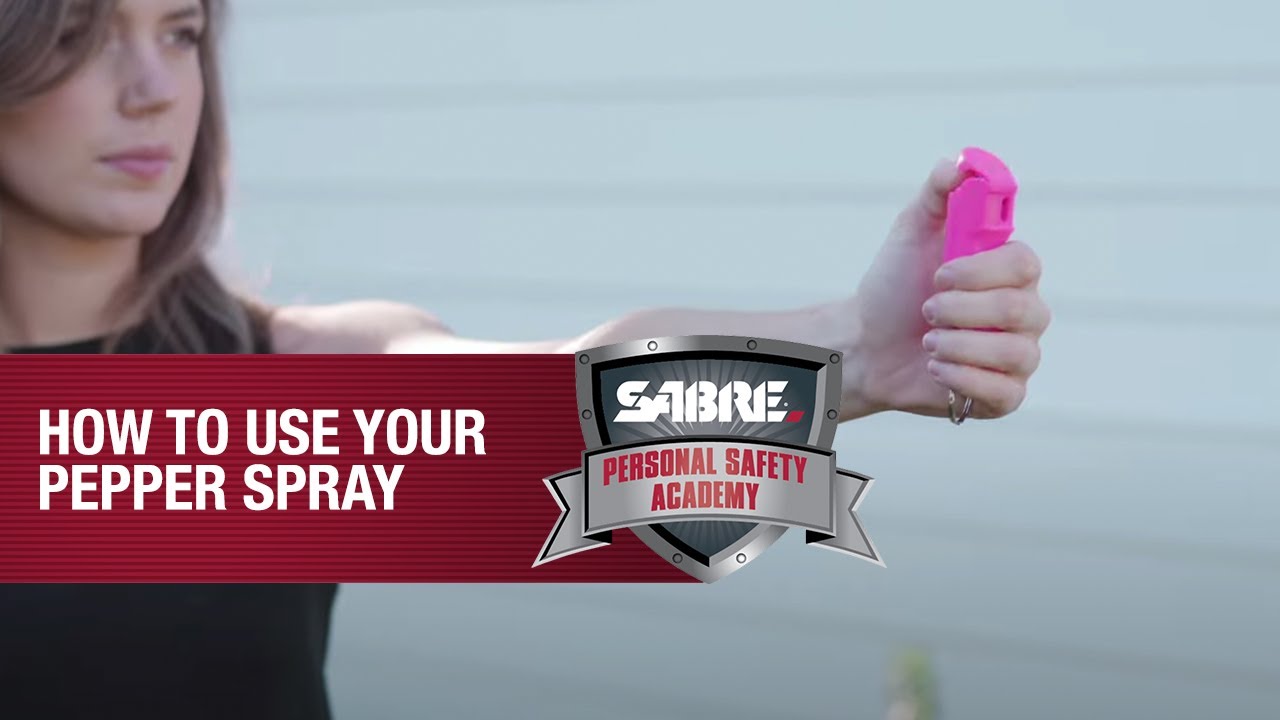In the image, which appears to be a promotional or instructional thumbnail, a woman in her 20s or 30s stands on the left side, holding a pink pepper spray canister. She is clad in a black sleeveless top with brown hair, and her left arm is extended to the right side of the image, poised as if ready to activate the pepper spray. Her backdrop is a house with white siding, slightly blurred. The pepper spray, held in a keychain-like case, is prominently featured. Across the bottom of the image, there is a red rectangular banner with white, all-caps, sans-serif font text stating, "HOW TO USE YOUR PEPPER SPRAY." Adjacent to this banner is a silver shield logo with a light gray sunburst design, displaying the word "SABRE" in white font. Below the shield is a forked gray ribbon with a red text that reads, "PERSONAL SAFETY ACADEMY."